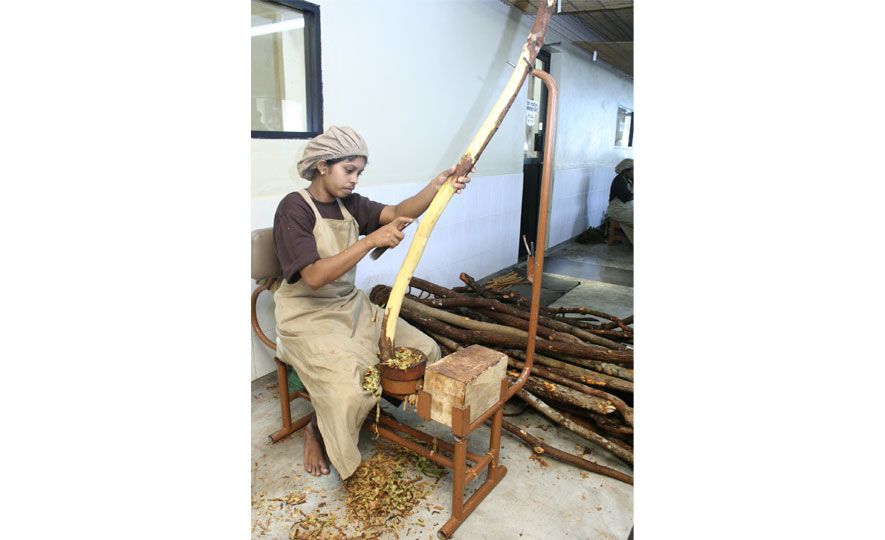The image portrays an Indian peasant woman meticulously removing bark from a large stick. Seated barefoot on a chair with a metal stand, the woman, dressed in a dark brown short-sleeve shirt and a light beige apron, uses a knife or a shaver to strip the bark. She is adorned with a hairnet and is working with a machine featuring a rod that curves upward, securing the stick in place.

Shavings accumulate in a nearby bowl and scatter across the concrete floor, creating a carpet of bark fragments. To her left lies a substantial pile of yet-to-be-debarked sticks, arranged on the ground. The setting is an indoor room with stark white walls, supplemented by black windows and a doorway in the background. Another worker, engaging in the same task, can be faintly seen to her left.